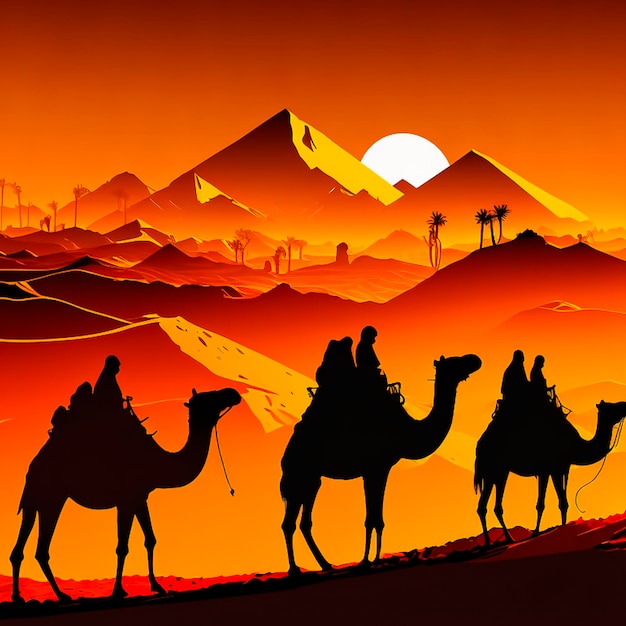This vivid piece of digital art portrays a sunset desert scene drenched in shades of orange, red, and yellow. In the foreground, three silhouetted camels traverse the sandy landscape from left to right. The lead camel, positioned farthest away, carries two riders, while each of the subsequent camels has a single rider. The silhouettes are stark black, emphasizing their mysterious journey. The background features rolling sand dunes and a scattering of palm trees, with five pyramids, the tallest positioned center-left, adding a touch of grandeur to the horizon. A bright white sun sets behind the pyramids, casting an orange hue that bathes the entire scene in warm light, enhancing the surreal and captivating atmosphere of the artwork.